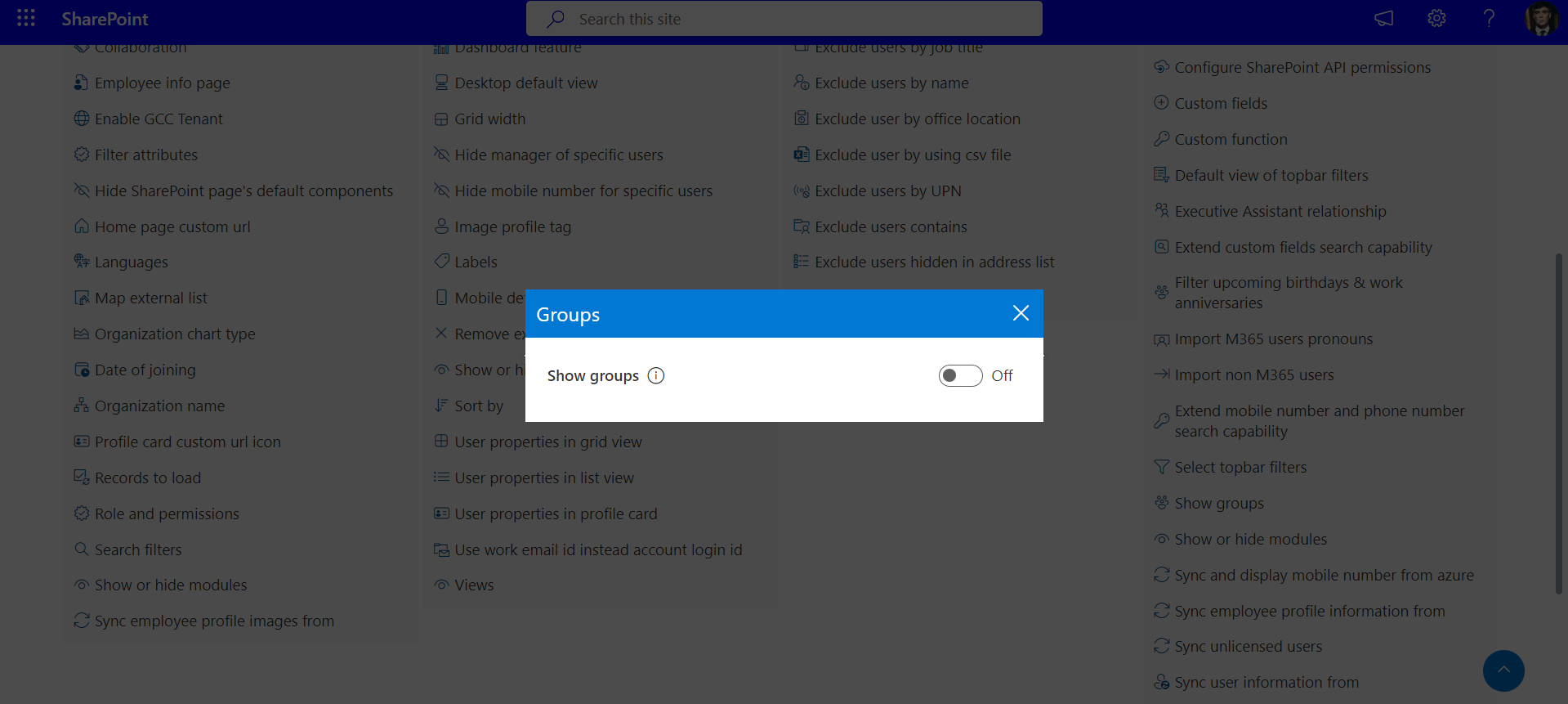The image features a SharePoint site interface with a semi-transparent overlay titled "Groups." The background of the overlay is blue, and it contains white text. In addition to the title, "Show Groups" is displayed prominently, with no items checked or selected. The underlying SharePoint page is visible but blurred, obscuring detailed content.